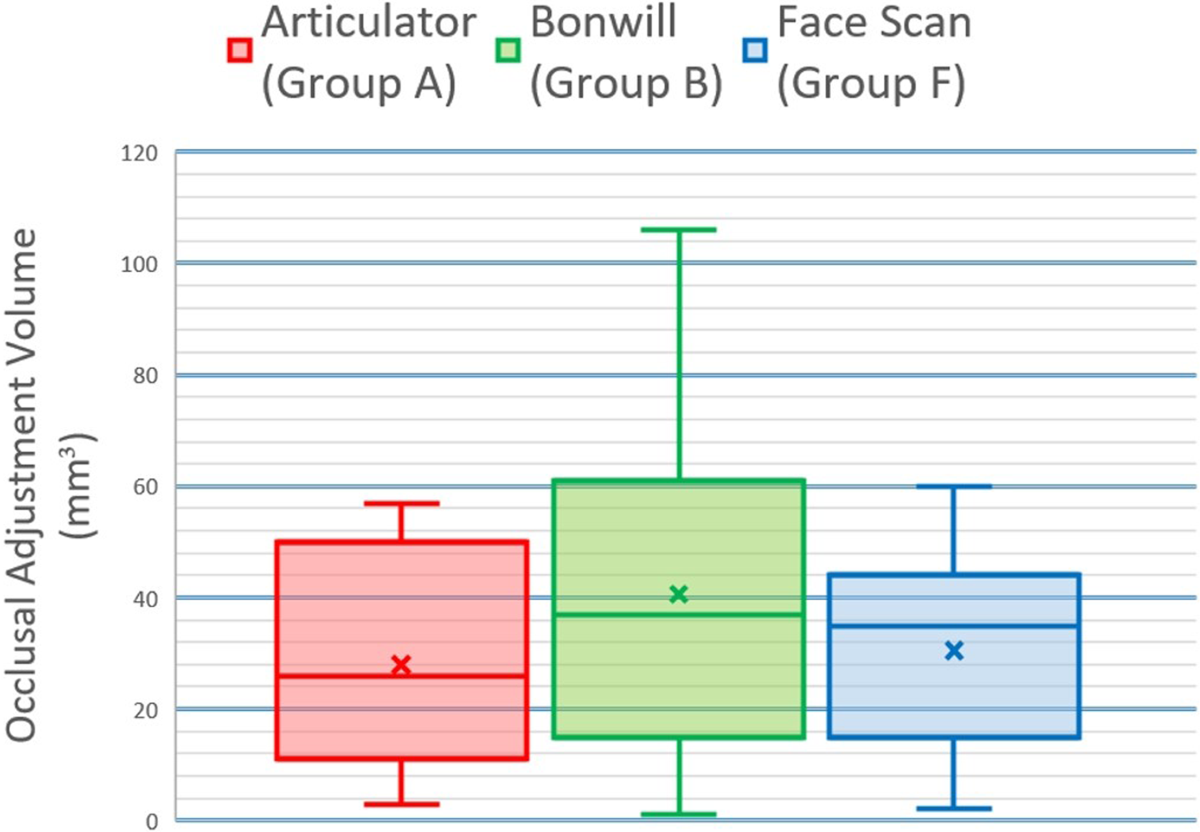The image is a detailed graph illustrating occlusal adjustment volume in cubic millimeters (mm³). The y-axis is labeled "Occlusal Adjustment Volume (mm³)" and ranges from 0 to 120 in 20-unit increments. Three groups are depicted using bar-like graphics in different colors, each with distinctive marking lines at the top and bottom. The red bar represents Articulator Group A, stretching approximately from 5 mm³ to around 58 mm³. The green bar, indicating Bonwill Group B, extends from the very bottom at 0 mm³ up to about 106 mm³, making it the highest. Lastly, the blue bar stands for Face Scan Group F, spanning roughly from 2 mm³ to 60 mm³. Each bar is marked with an X at specific points to highlight key values. The white background provides a clear and clean context for the data displayed.